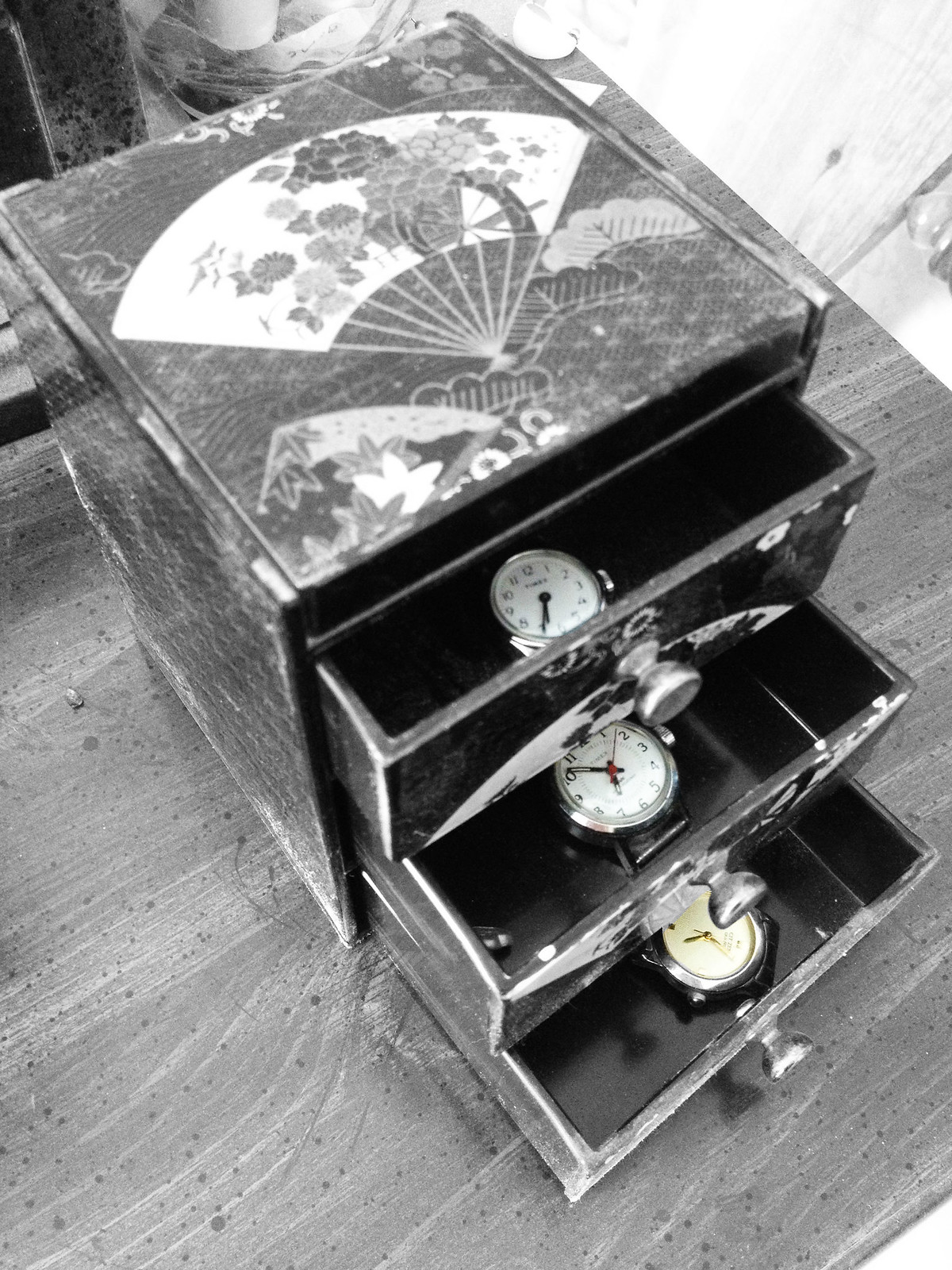This black and white photograph of an antiquated piece of furniture is meticulously captured with certain details in color, forming a striking contrast. The chest of drawers, potentially a jewel box, showcases three slightly open drawers, each housing a distinct pocket watch at its center. These pocket watches are of different makes and styles but share a similar size. The top drawer contains a reflective metal watch with visible numbers and black minute and hour hands, underlining its subtle color amidst the grayscale. The middle drawer holds a pocket watch with a white face, complete numbers, a white minute and hour hand, as well as a red second hand. The bottom drawer, which extends the furthest, features a hexagonal pocket watch with a yellow face and gold hands, marked only by a dot representing 12. The box itself, likely made of worn leather, is adorned with a delicate Japanese-style fan graphic on its top, embellished with flowers, hills, valleys, and possibly trees, adding an intricate artistic touch. A Victorian-clad woman’s image subtly peeks through these designs. This entire setup rests on a beautifully textured hardwood table, its detailed patterns complementing the antique nature of the chest. Silver knobs accentuate the drawers, and there are nondescript items in the background, barely discernible due to the black and white filter.